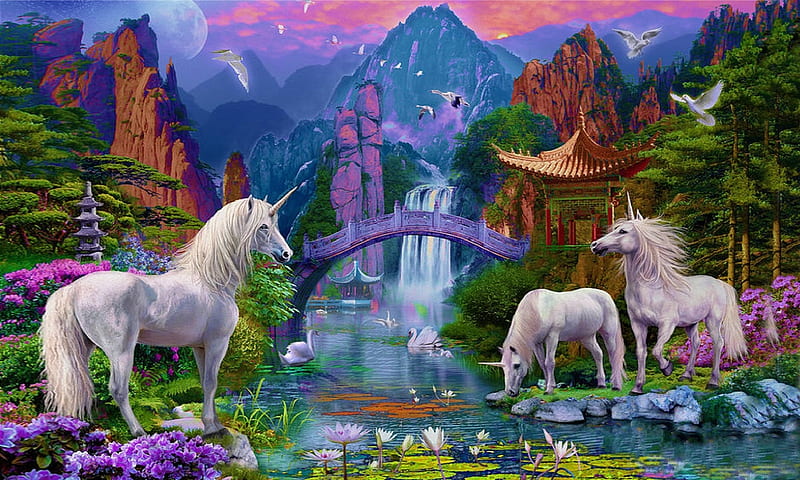This vibrant digital artwork captures an enchanting, fantasy scene dominated by a central stream adorned with green lily pads and pink flowers. The stream winds its way from a distant waterfall cascading down a steep, dark gray mountain peak. The sky above the mountains is a mesmerizing blend of lavender, violet, orange, red, and yellow hues, depicting a breathtaking sunset, with a pink-clouded sky transitioning into dusk along with a faint moon glow.

In the foreground, on the left bank of the stream, a lone white unicorn with a majestic white mane and tail stands amid a bed of purple flowers. Behind it, a cluster of pink and blue flowers surrounds a small stone statue resembling a four-tiered spiked house. To the right, closer to the stream, a pair of white swans gracefully glides on the water. 

On the right bank of the stream, two unicorns, also white, bring additional life to the scene—one lowering its head to drink, while the other stands elegantly with its mane and tail animated as if caught in a gentle breeze. Behind them, bushels of pink flowers dot the green grass, creating a picturesque setting. 

Further enhancing the fantasy ambiance, an architecturally intricate purple bridge arches over the stream, leading to an Asian-style temple with a distinctive flared roof situated on the right side. Additional elements include scattered pink flowers and pine trees creating a serene backdrop, with white doves and various other birds soaring above.

A little shrine, similar to the temple but smaller, is nestled among flowers on the left side, providing symmetry to the meticulous details of the artwork. The entire scene, contained within a rectangular frame approximately 5 to 6 inches wide and 4 inches high, exudes a serene yet magical atmosphere, immersing the viewer in a breathtaking convergence of nature and mythical creatures.